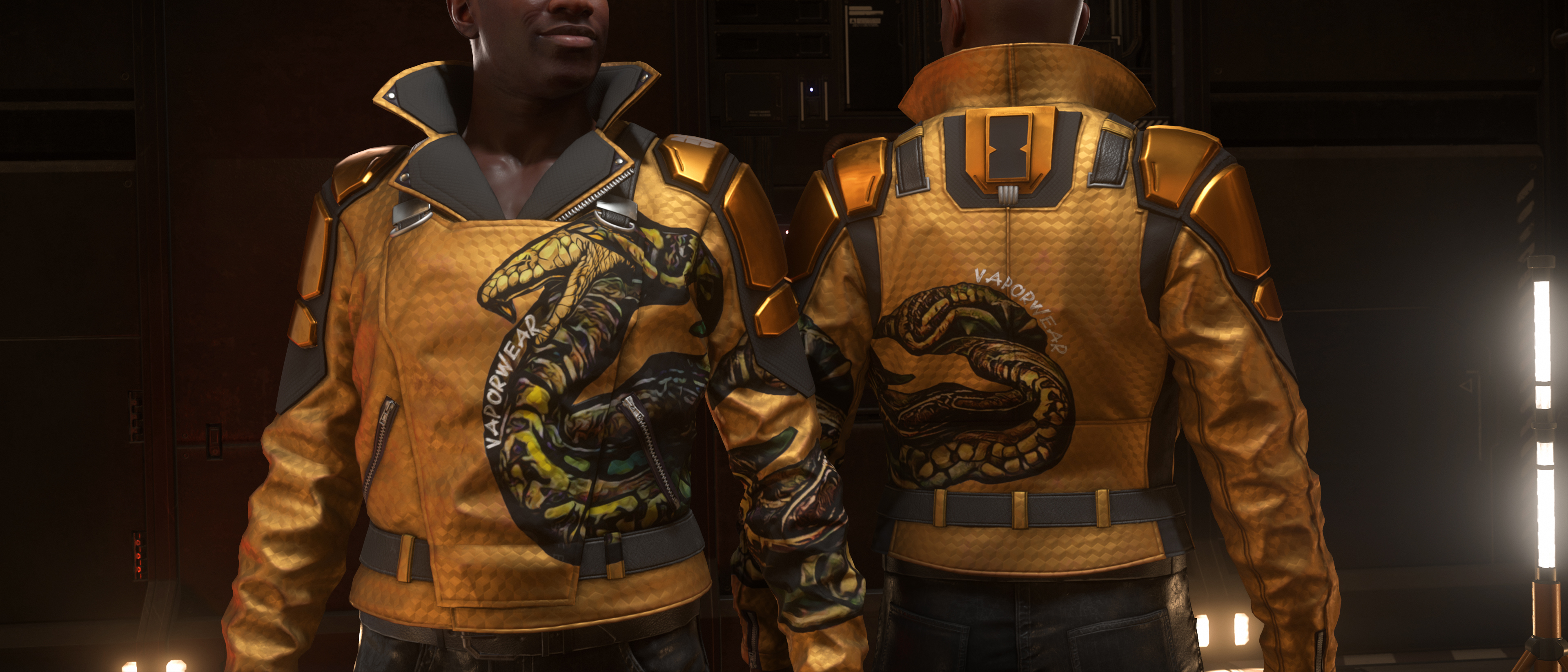The photograph features a prominently displayed, stylish black and gold jacket adorned with an intricate snake design. The snake's head and body start on the front right side of the jacket, extending from the bottom of the abdomen slithering up to the left. This serpentine design continues seamlessly onto the back of the jacket. The image shows two figures: one facing forward, allowing us to observe the front of the jacket; and another standing with their back towards us, revealing the snake's continuation onto the back of the garment. The second figure enables a full view of the snake, showcasing its tail and lower end on the back right side. The jacket is a coppery gold color with subtle touches of black and yellow, exuding a rock star aesthetic reminiscent of a piece worn by Michael Jackson. The scene is set in a dimly lit room with a lot of black and darkness in the background, adding to the dramatic presentation. Additionally, the forward-facing figure has a belt, gray in color, accentuating the waist. The photograph is meticulously curated to provide a comprehensive view of the elaborate jacket, from the front and the back.